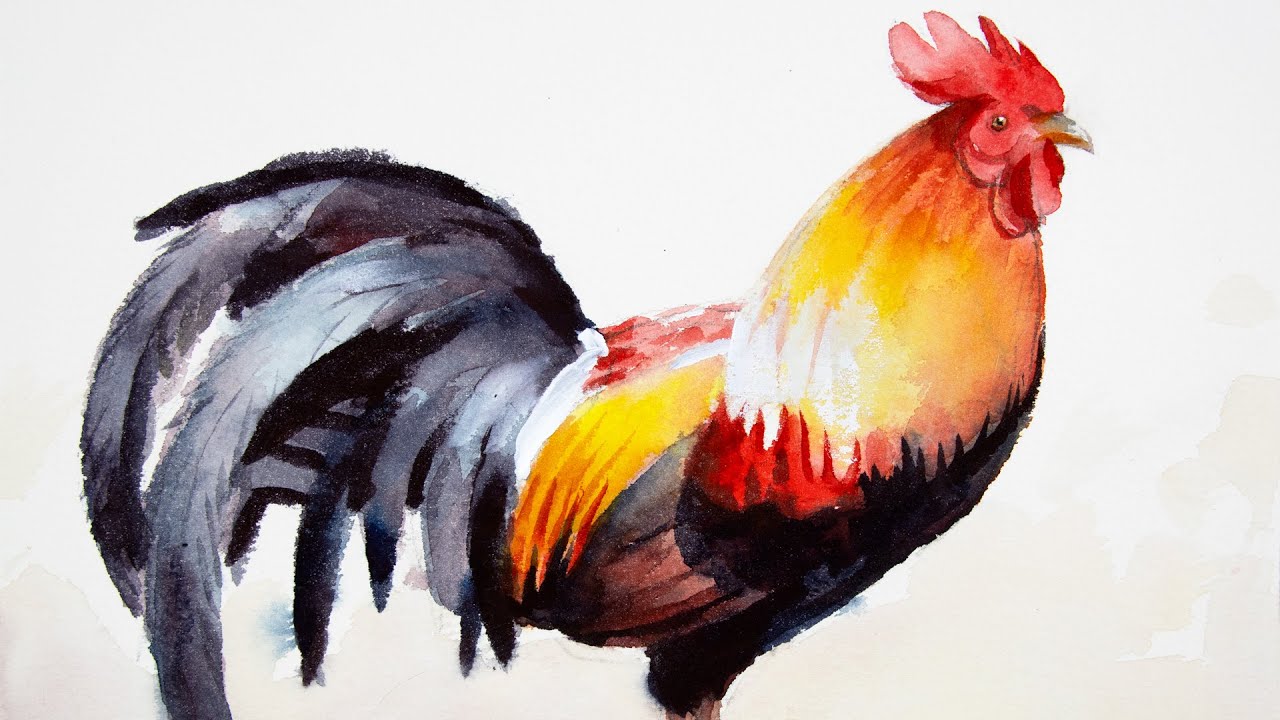This painting captures a proud rooster rendered in watercolor, standing out vividly against a white, unsigned background. The rooster’s vibrant plumage transitions from a fiery red head to a mix of orange, yellow, and white feathers cascading down its neck and torso. The lower body feathers eventually shift to a dark, almost purple hue, and the strong, black-feathered legs. The tail feathers are expansive and flamboyant, predominantly black with hints of blue and white to suggest a glossy sheen. The rooster’s head features a pronounced red mask and face, with piercing black eyes and a gray-toned beak. The overall composition emphasizes the rooster's majestic and confident stance, making it a striking focal point.